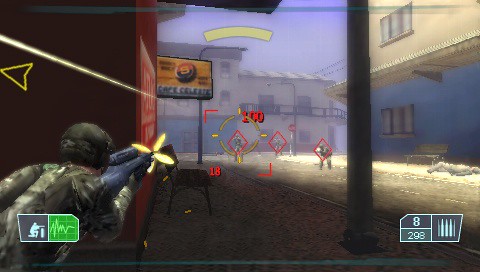A screenshot captures intense action from a video game, possibly a first-person or third-person shooter. Dominating the left side of the screen is a soldier clad in camouflage, engaged in a firefight while aiming a weapon that appears to be either a sniper rifle or an assault rifle. This soldier is firing at enemy combatants positioned in the distance. The game's HUD (Heads-Up Display) in the bottom left corner features an icon of a soldier in a kneeling position, accompanied by a green heartbeat line, suggesting health status. Additionally, numerical readings next to this icon display "8" and either "293" or "298." Another indicator shows bullet icons, likely representing the remaining ammunition.

The backdrop reveals an urban setting resembling a third-world country's downtown area. A prominent billboard displays the words "Cafe Submarine" alongside an icon and the number "9." Visible in the distance are three enemy combatants, each marked with red diamond-shaped indicators, highlighting them as targets. Various sight marks and reticles are also present, aiding the player in aiming. The overall color palette of the scene includes beiges, reds, blues, and the distinctive camouflage pattern on the soldiers, contributing to the immersive atmosphere.